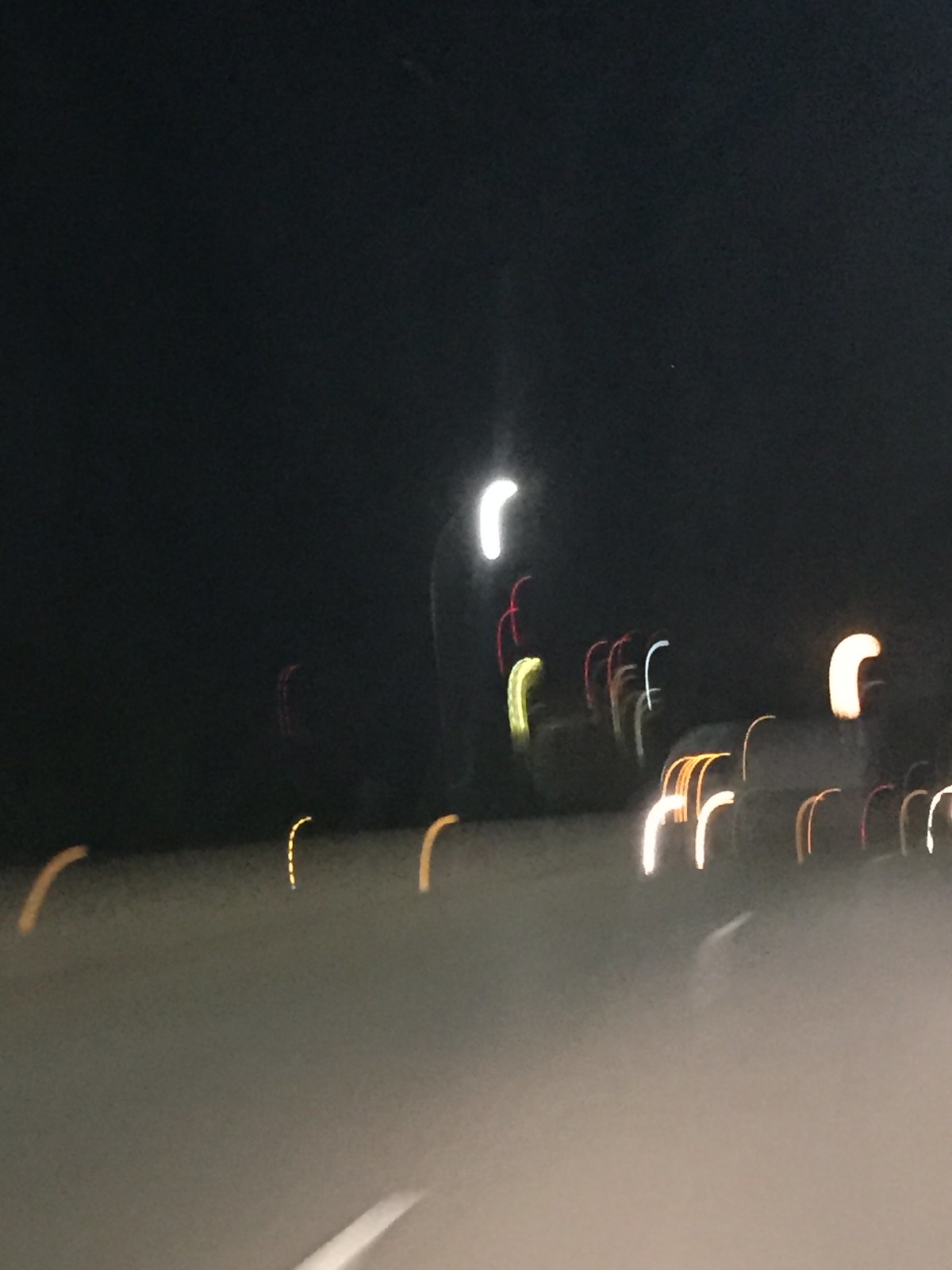This color photograph, taken at night, captures a blurry scene from the perspective of a moving vehicle. The majority of the top two-thirds of the image is enveloped in a deep black darkness, providing a stark contrast to the colorful lights scattered below. These lights appear as thick and thin cane-shaped streaks in hues of white, orange, blue, red, and yellow, likely due to the camera's movement during the shot. The lights cluster predominantly in the middle of the photo, stretching from the left side to the right with fewer lights dispersed on the outer edges. Below the vibrant display of lights, the lower part of the image transitions to a grayish blur, resembling a road with visible white dashed lines indicating lanes. The road tapers off into the distance, bordered by what appears to be a rounded, grassy roadside. The scene captures the surreal and distorted reflections from the vehicle's dashboard and other surrounding lights, creating an abstract and dynamic nighttime landscape.